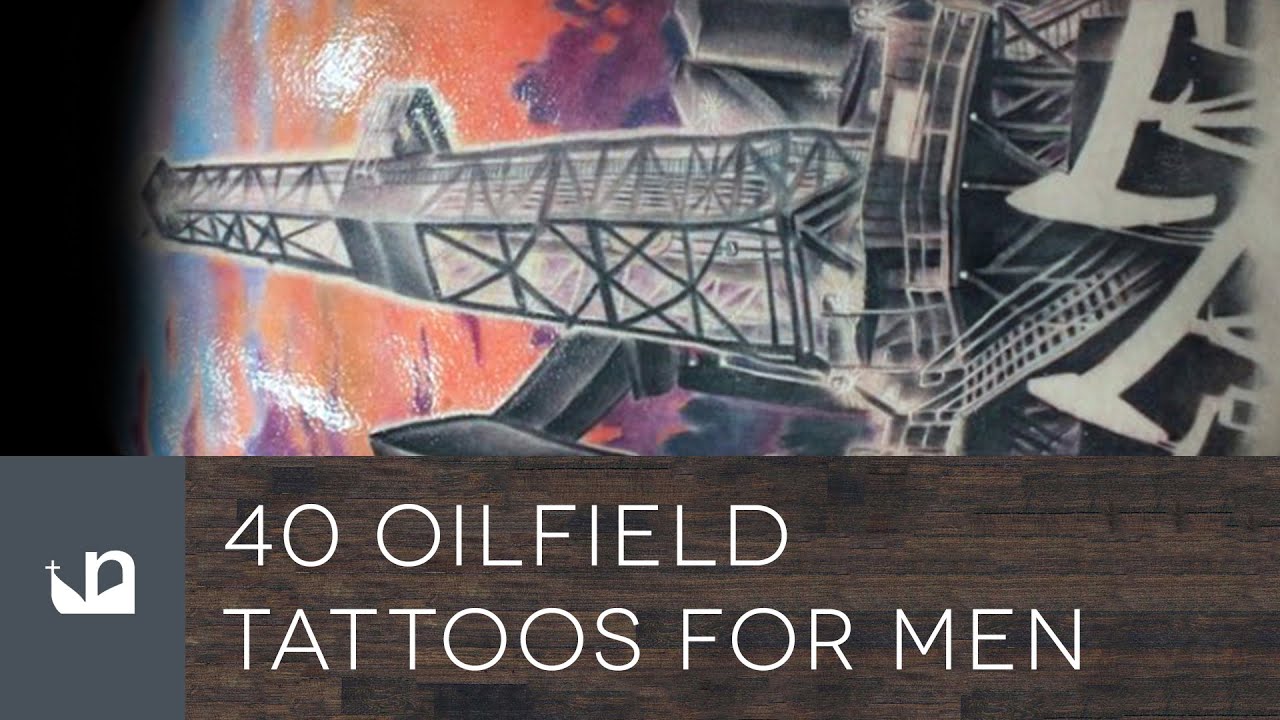This image likely serves as an advertisement, possibly for a website, video, or product related to oilfield tattoos for men. The overall layout is in landscape orientation and is divided into two main sections. The bottom third features a wood-grain patterned background with white text that reads "Forty Oilfield Tattoos for Men." On the left-hand side of this wooden section is a gray box containing a white logo that appears to be an open book with a lowercase 'n' and elements resembling leaves and a cross. 

The top two-thirds of the image showcase a detailed, horizontally-oriented tattoo design depicting an oilfield. At the center, there is a prominent black and white image of a steel-framed oil derrick tower lying sideways, surrounded by various oil pump jacks typically used to extract oil from the ground. The background of the tattoo features a vibrant sunset sky with a color gradient ranging from blue to orange to a mauve-like purple. Additionally, scattered across the image are hues of orange, magenta, and blue, enhancing the picturesque scene. The overall image has a glossy, almost shiny appearance, giving it a realistic and striking visual impact.